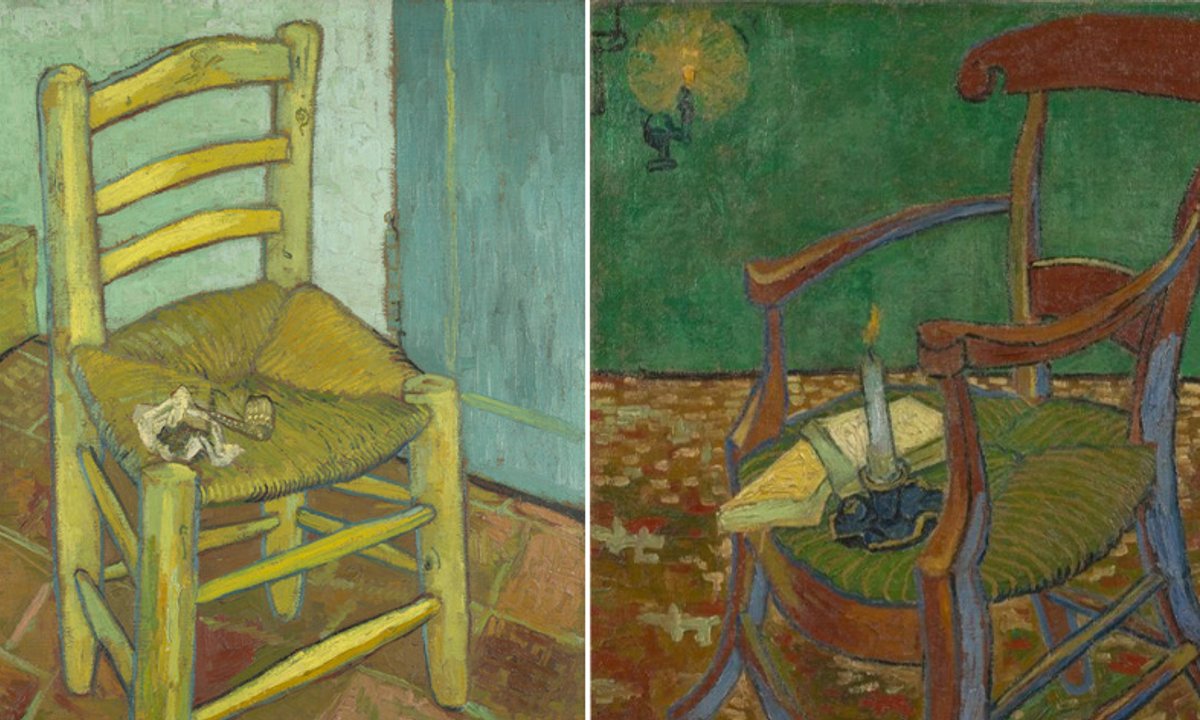This rectangular image, approximately 6 inches wide and 3 inches high, showcases reproductions of two iconic paintings side by side, separated by a thin white vertical line. The left painting is Vincent Van Gogh's "Chair," depicting a rustic, yellow wooden chair grounded on red brick tiles. The chair features a woven straw seat with four sections meeting in the center in an X pattern. Small unidentified objects rest on the seat. The background is a divided wall, light blue on one side and a darker blue-green on the other, separated by a corner seam.

In contrast, the right painting is Paul Gauguin's "The Armchair," illustrating a dark wooden chair with armrests. The chair similarly has a woven wicker seat. A lit candle in a dark metal holder and two small books share the seat. The floor beneath is patterned, resembling a carpet with leaves in shades of brown, yellow, and red. The background reveals a dark green wall with a subtle light sconce, emitting dim orange light.

Both paintings capture the essence of their artists' unique styles, linked thematically by the presence of chairs, yet differing in color palettes, chair designs, and environmental details.